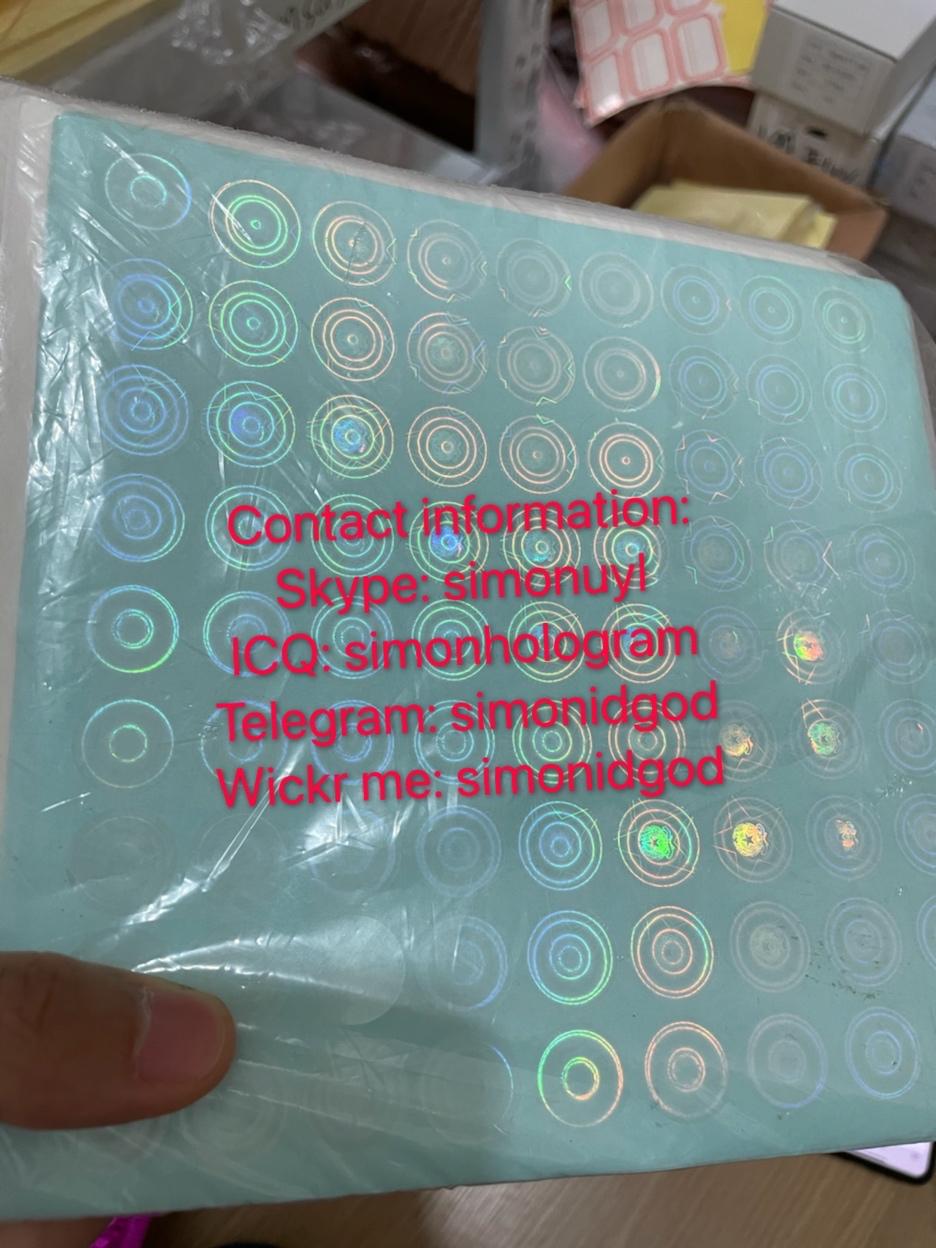In this image, only the thumb of a person is visible as they hold an aqua blue square piece of plastic encased in a transparent polythene bag. The plastic features an elaborate, colorful pattern consisting of numerous metallic, color-changing circles arranged in a grid, with about ten circles per row and column. Each circle has intricate designs, with some containing one or more concentric circles inside them. The background reveals a floor setting strewn with various daily items including boxes, file folders, and stickers.

Prominently displayed in red text over five lines on the plastic are multiple contact methods for someone named Simon: "Contact Information: Skype: SIMONUYI, ICQ: SIMONHOLOGRAM, Telegram: SIMONIDGOD, Wicker Me: SIMONIDGOD." The lower part of the image shows a brown desk or table beneath the item being held, completing the scene.